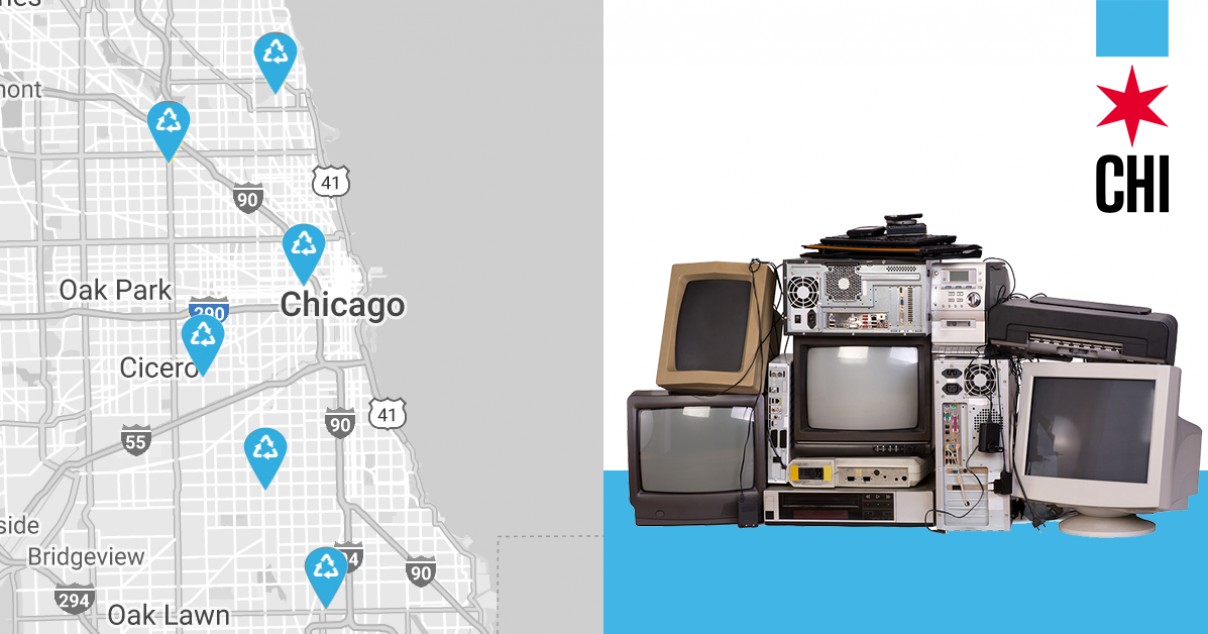The image has two sections: the left side features a detailed map of the Chicago area highlighting neighborhoods such as Oak Park, Cicero, Bridgeview, and Oak Lawn, with major highways like 90, 41, 55, and 294 prominently marked. The map includes a light gray land representation and a distinctive gray area for Lake Michigan. Scattered throughout the map are blue pear-shaped symbols, potentially indicating recycling centers. The right side showcases a heap of outdated electronic equipment, including computer monitors, TV screens, VCRs, and possibly old CPUs, all set against a background that transitions from blue at the bottom to white at the top. The upper right corner features a light blue square with a red star and the letters "CHI," reminiscent of the Chicago city flag's colors and elements. The combination of the two images, along with the recycling symbols, suggests the promotion of electronic recycling initiatives in the Chicago area.